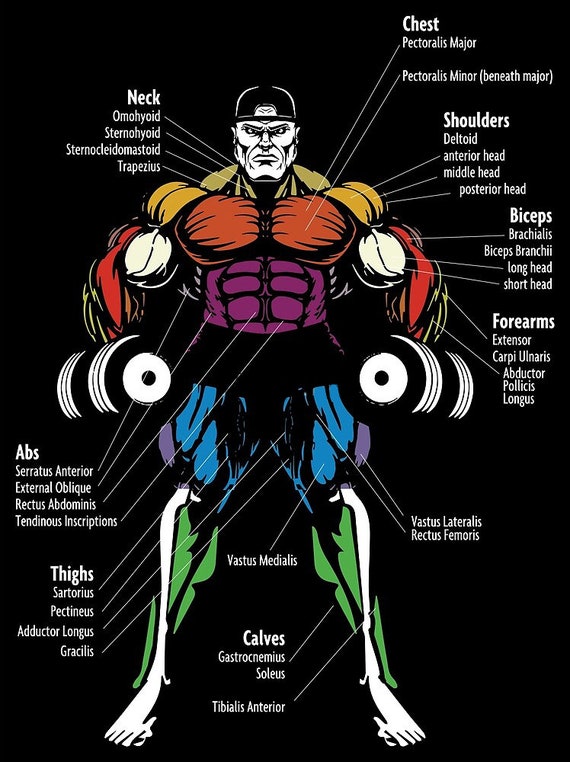This image is a highly detailed infographic or schematic poster of a very muscular, cartoon-like bodybuilder who is holding two dumbbells, one in each hand, with his legs apart. The bodybuilder is shirtless and pantless, wears a backwards black cap, and stands against a completely black background. Various muscle groups across his body are highlighted in different colors to differentiate each muscle group: green for the lower legs, blue for the thighs, purple for the outer thighs, orange for the chest, yellow or golden for the shoulders and traps, and red for the biceps and arms. Muscles are outlined clearly, with the major muscle groups distinctly marked and labeled. Each muscle group label is in bold with the detailed names of individual muscles listed underneath in smaller script. For example, the chest muscles are labeled as "chest" with terms like pectoralis major and pectoralis minor indicated underneath. Similarly, the abdominal area includes detailed labeling of muscles such as the serratus anterior, external oblique, rectus abdominis, and tendinous inscriptions. This comprehensive and colorful diagram serves as a training tool, likely intended for educational purposes within the medical or physiotherapy fields.